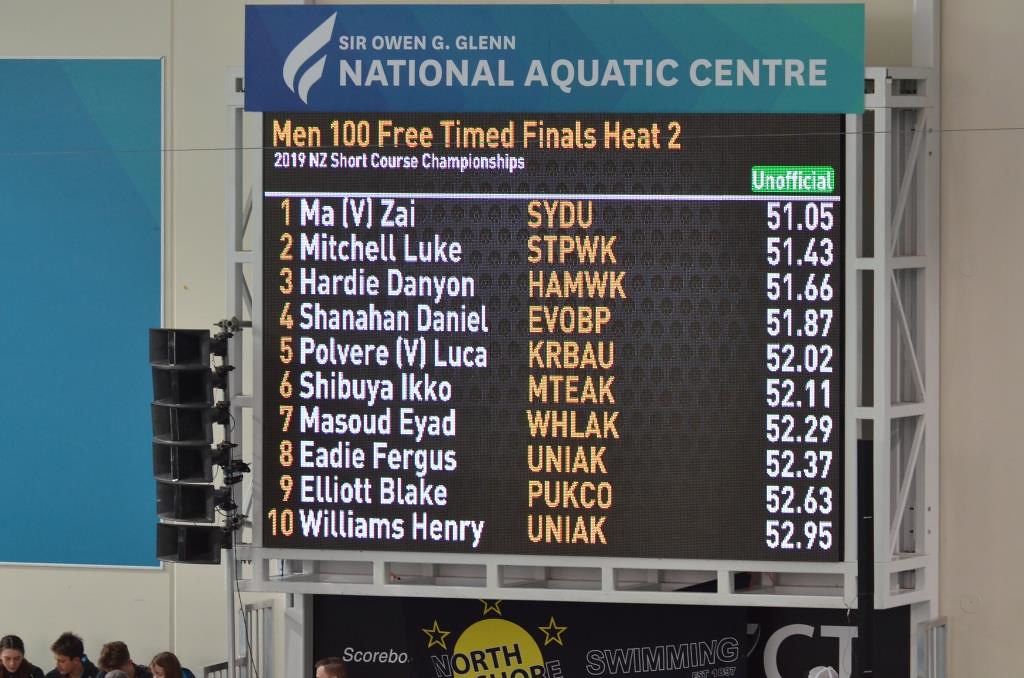The image depicts a large scoreboard at the Sir Owen G. Glenn National Aquatic Center during the 2019 NZ Short Course Championships. The scoreboard prominently displays the results for the Men’s 100 Free Time Finals Heat 2, with the names of the top 10 finishers and their respective unofficial times. The first place was Ma Zhao from SYDU clocking in at 51.05, followed by Mitchell Luke from STPWK with a time of 51.43. Other competitors include Hardy Dannion, Shannon Daniel, Palavra Luka, Shibuya Iko, Masood Iyad, Edie Fergus, Elliot Blake, and Williams Henry. The scoreboard features a distinctive design, with a half dark blue, half lighter blue or greenish header, and a small green box to the right indicating the times are unofficial. Below the scoreboard, there's a visible advertisement for a swim event, and the heads of several spectators can be seen in the foreground. The background wall is white.